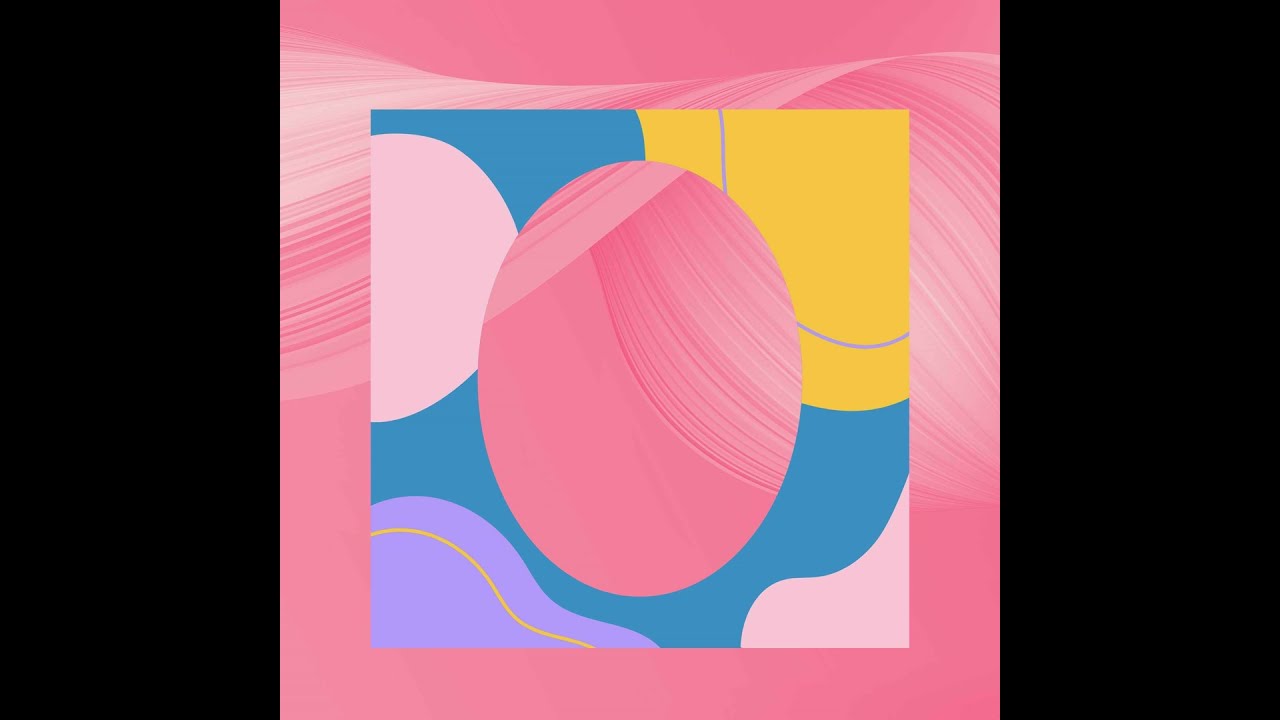This artistic piece features a horizontally rectangular design with thick black borders on both the left and right sides, while the top and bottom remain borderless. At the center, a large pink square dominates the composition, adorned with flowing, wavy white lines that create a ribbon-like effect, reminiscent of hair etching. Inside this pink square is another vibrant square filled with a mosaic of multiple colors including blue, yellow, white, and various shades of pink, as well as teal, gray, and violet. In the very middle of these layered squares, there's an egg-shaped pink figure with striations and stripes, highlighting the design’s complexity. This central egg shape is surrounded by abstract, swirling patterns, creating an intricate, almost symbolic visual narrative that blends hand-drawn and possibly digital artistic elements.